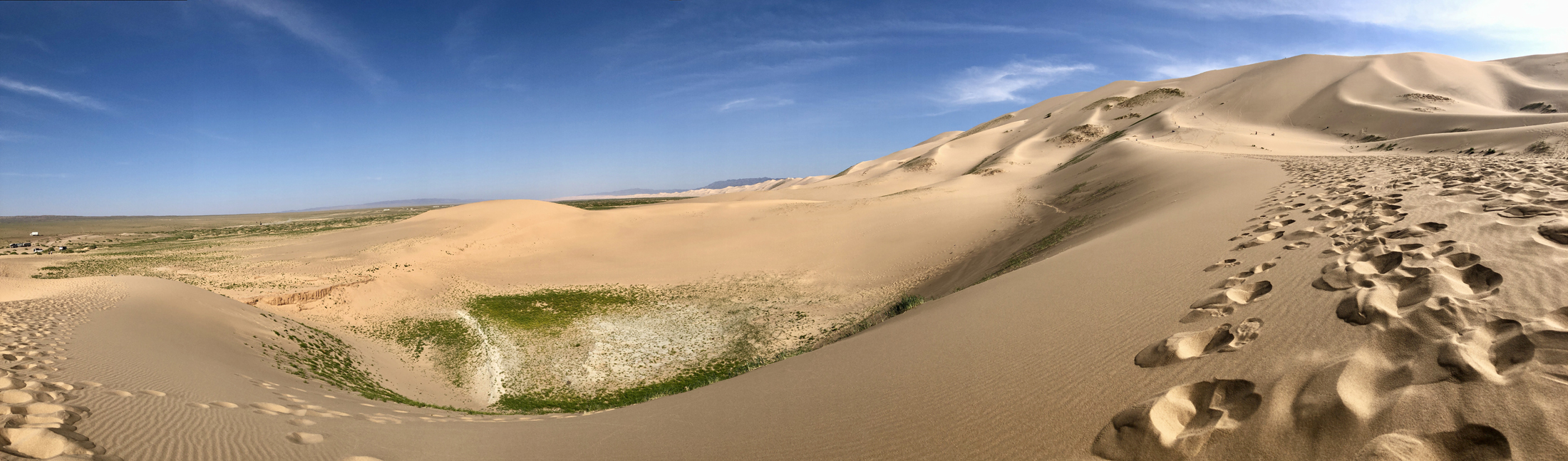This is a full-color outdoor photograph taken on a bright, sunny day, depicting an expansive landscape of sand dunes under a vivid blue sky with a few wispy white clouds. The upper part of the image is dominated by the blue sky that extends from the left to the center with some clouds appearing towards the right. The desert terrain, characterized by its sandy hills, features prominently in the foreground and mid-ground.

To the right side of the image, there is a large sand dune with multiple indents indicating where people or possibly large animals have walked, moving slightly uphill towards the upper right corner. The bottom right corner also shows distinct footprints, likely shoe prints, embedded in the sand.

In the left foreground, a slight valley in the sand houses patches of green vegetation, including grass shrubs. Additional patches of greenery are visible slightly left of center and further into the distance, suggesting some presence of plant life amidst the arid environment.

The color palette of the image ranges from beige and brown tones of the sand to the light and dark blues of the sky, accented by whites and some dark elements possibly from shadows or deeper footprints. The overall impression is a serene, natural scene highlighting the interplay between the clear sky and the undulating sand dunes, with subtle hints of life persisting in the harsh desert landscape.